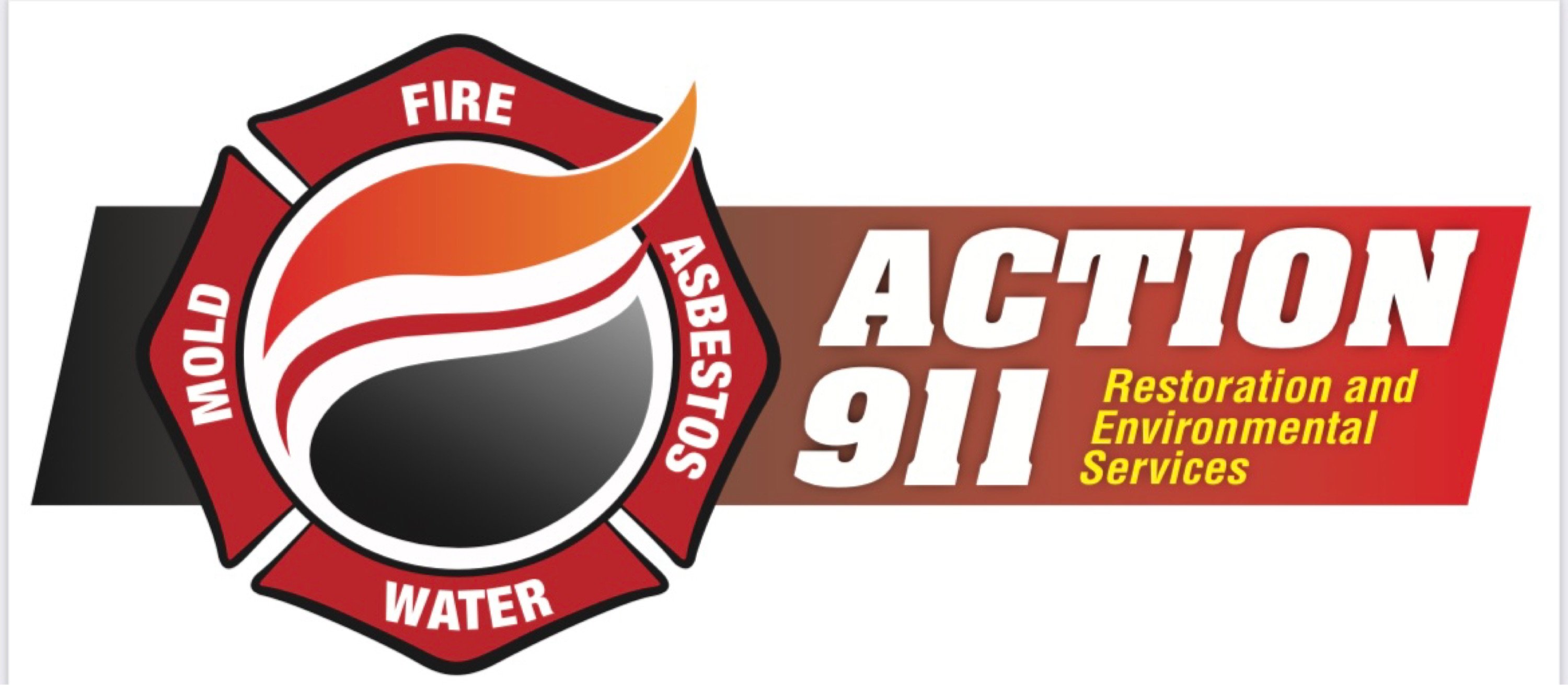The logo prominently features a horizontal banner that transitions from red on the right to dark gray on the left. Centered on the left portion of the banner is a circular, shield-like emblem. This emblem contains an image of a flame, with the flame subtly extending to the right side of the circle. Encircling the flame within the emblem are the words: "Fire," "Asbestos," "Water," and "Mold," representing different hazards.

To the right of this shield, the banner displays the company's name and services. The text "Action 9-1-1" appears in bold white letters, while "Restoration & Environmental Services" is written in vibrant yellow. The overall design combines a modern gradient background with elements symbolizing safety and emergency response.